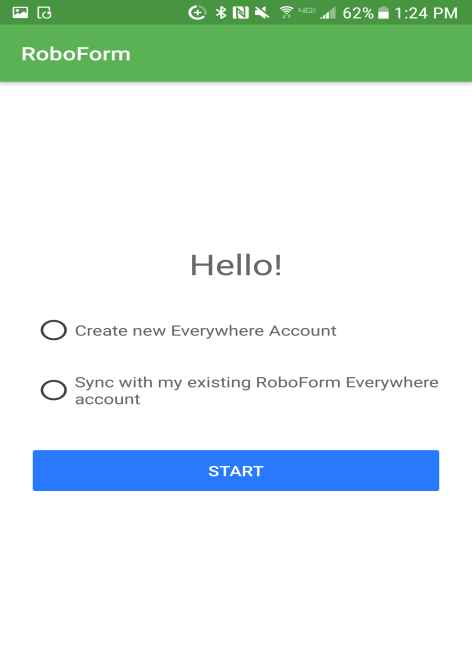A detailed and cleaned-up descriptive caption for the image:

The image is a screenshot of a small document or form displayed on a mobile phone screen. The background of the form is white, with a green header and footer. At the very top of the screenshot, there is a thin green bar displaying various status icons. 

On the right side of this bar, the time is shown as 1:24 p.m. Next to the time is a battery icon indicating 62% charge remaining. There are also icons for Wi-Fi (showing three bars of signal strength), Bluetooth, and other standard phone indicators. On the left side of the green bar, there are additional icons, including one for photos. 

Directly beneath this green bar, centered, is the text "RoboForum," suggesting the name of the form or application. The body of the form contains ample white space, followed by a greeting that reads "Hello." Below this greeting are two options presented with circular checkboxes to the left of each option. The first option reads "Create new Everywhere account," and the second option reads "Sync with my existing RoboForum Everywhere account." 

At the bottom of the form, there is a prominent blue button labeled "Start."